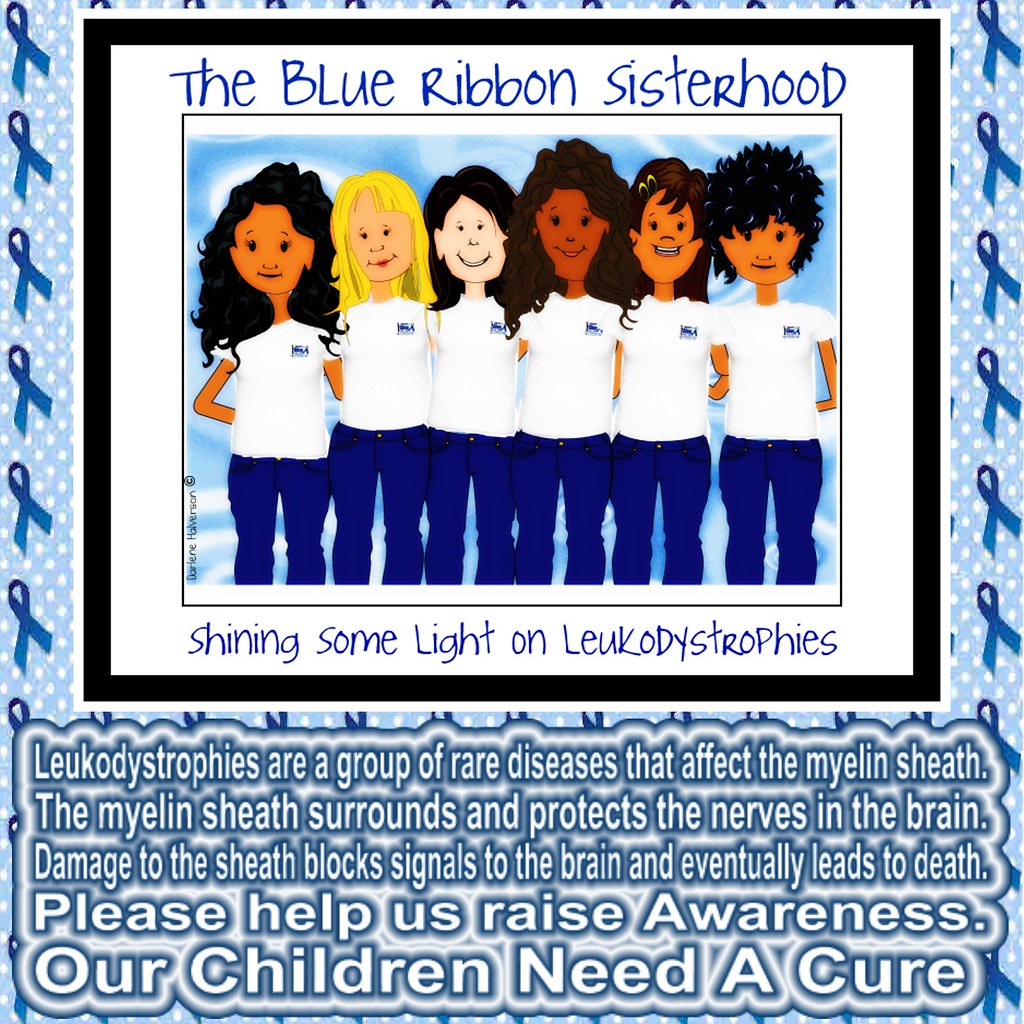The image depicts an artistic, cartoon-style representation of the "Blue Ribbon Sisterhood," framed in a black box against a white background. The top features blue text reading "The Blue Ribbon Sisterhood," while the bottom contains the phrase "Shining some light on Leukodystrophies." The illustration shows six women of various races, each wearing white shirts and blue jeans, standing arm-in-arm. The women are diverse, with different skin tones and hair colors, including black and blonde hair, and brown and white skin. The background is blue with white polka dots and blue ribbons along either side. Below the cartoon, informative text in white letters, outlined in blue, explains that Leukodystrophies are a group of rare diseases affecting the myelin sheath, which surrounds and protects the nerves in the brain. Damage to this sheath blocks signals, eventually leading to death. The caption concludes with a plea: "Please help us raise awareness. Our children need a cure."